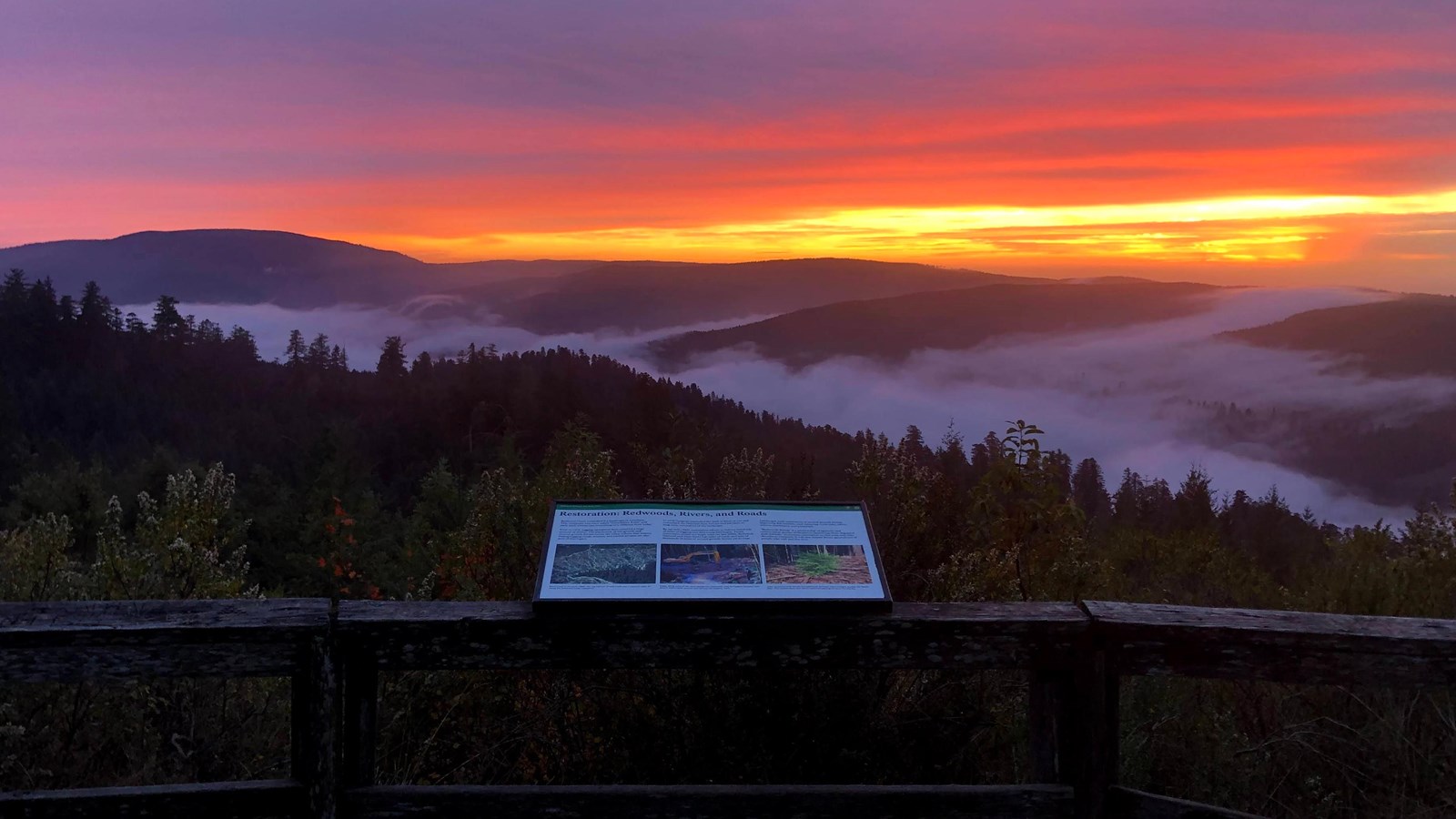This captivating outdoor photograph captures an overlook area with a wooden barrier at the forefront, where a framed informational sign is perched on a concrete ledge, although the text remains unreadable from this distance. The viewpoint reveals lush green trees descending into a fog-blanketed valley, leading to a majestic mountain range in the distance. The sky is awash with stunning hues of red, orange, yellow, and purple as a mesmerizing sunrise—or possibly sunset—paints the clouds with vibrant colors. The early morning mist adds a mystical aura to the serene landscape, further enhancing its beauty.